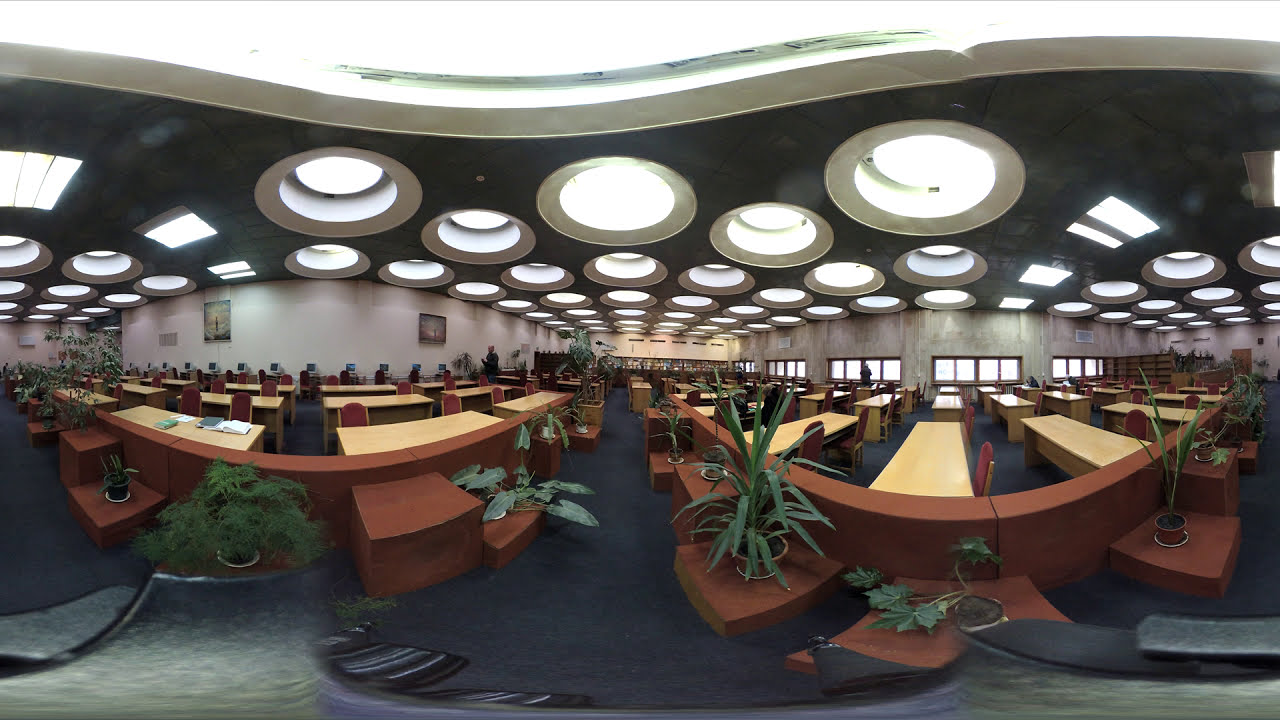The photograph is a panoramic view of a vast indoor space that likely serves as a conference center or a large office setting. The ceiling is a distinctive feature, characterized by its curved form and an array of circular and square skylights that allow natural light to flood the area. Dark gray in color, the ceiling also contains recessed lighting arranged in no particular pattern.

The layout below the ceiling is lined with a mix of brown wood furniture and long, light brown tables accompanied by dark red chairs. Desks can be seen running both horizontally and perpendicularly along the curvature of the walls, which are a long brown color and feature windows with brown frames on the right side and paintings on the left.

Adding a touch of nature, dark green indoor plants are spread out randomly throughout the floor space, bringing a sense of freshness to the scene. The flooring is covered in a navy blue carpet, creating a cohesive color scheme when combined with the other elements in the room.

The overall setting is well-lit, likely by the natural daylight coming through the skylights, giving the impression of a bright and welcoming environment. The objects in the room are positioned evenly across the space, contributing to an organized and spacious appearance.